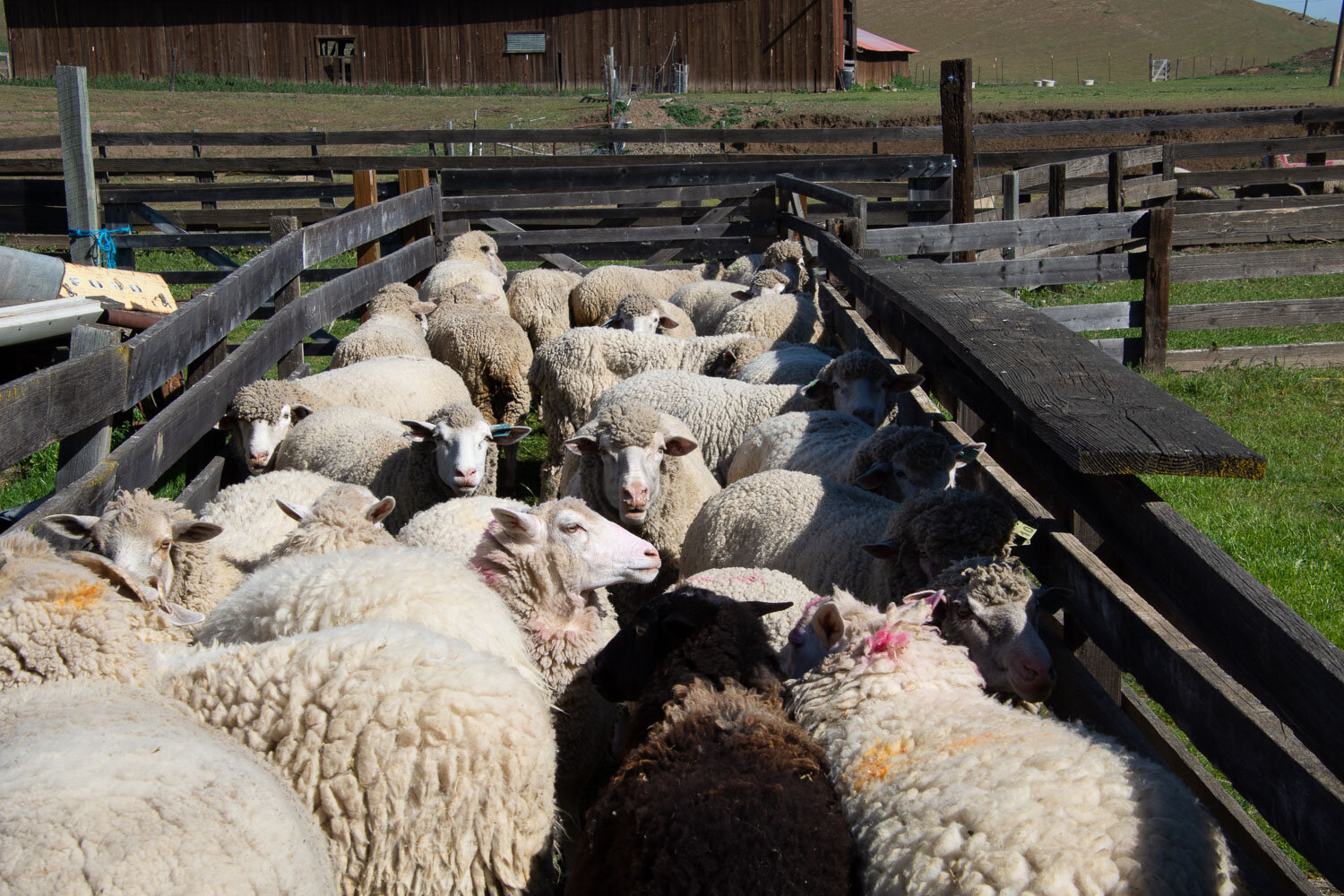This detailed, overhead color photo captures an active farm scene bathed in sunlight. Central to the image is a bustling lane lined with weathered, gray wooden fences, guiding a herd of approximately 20 sheep towards an open corral. The sheep, predominantly white and gray, with one notable black sheep and another brown one, appear mature with full, un-sheared coats. They are bunched together, with a few looking towards the camera, though most gaze away. Surrounding the lane, there's a backdrop of lush greenery and grass. Dominating the horizon is a large, rustic brown barn, alongside a smaller yellow building topped with a red awning. To the side, some farm equipment is partially obscured. A sliver of blue sky peeks from behind a hill in the upper right corner, highlighting the summer day ambiance.